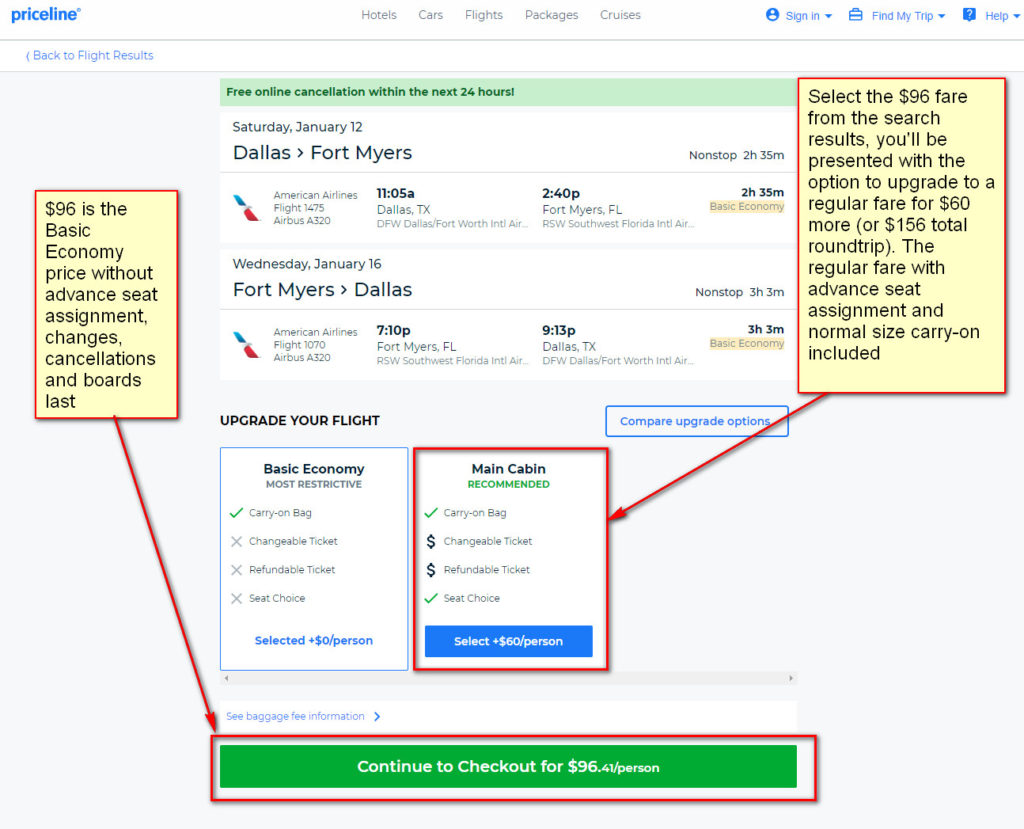Screenshot from the travel booking website, Priceline, highlighting the different fare options for a round trip flight from Fort Myers to Dallas. The screenshot showcases various on-screen elements including:

- Headings such as "Free Online Cancellation," "Sign In," "My Trips," and "Help" at the top.
- A fare selection section where the $96 basic economy option is emphasized. This fare does not include advanced seat assignments and has restrictions like no changes, no cancellations, and boarding with the last group.
- A detailed option to upgrade to regular fare for $60 more, totaling $156 for the round trip. This fare includes advanced seat assignments, a normal-sized carry-on, and main cabin privileges.
- Interactive buttons for proceeding with the purchase: a green "Continue to Checkout" button for the basic economy fare, and a blue "Select Main Cabin" button for the upgraded fare.
- Visual highlights including a red box and arrows pointing at the main cabin fare option and the continue to checkout button, guiding the user’s attention towards these options.

This detailed screenshot serves as an informative guide for users comparing fare options and making their selection on the Priceline website.